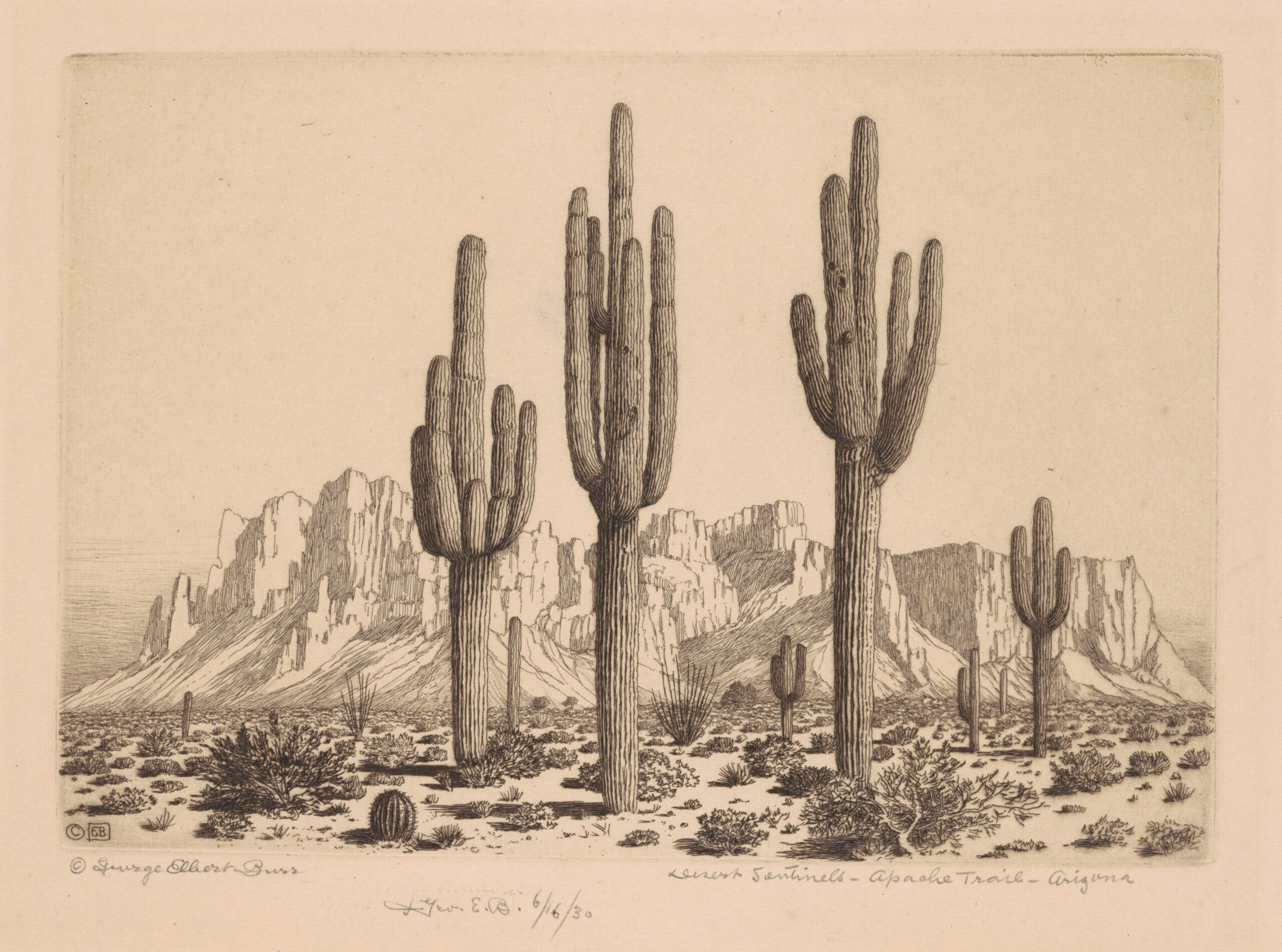The image depicts a detailed and textured hand-drawn desert landscape, likely situated along the Apache Trail in Arizona. Dominating the scene are three large cacti centered prominently, accompanied by an additional two cacti positioned to the right. The ground, primarily occupying the lower portion of the image, showcases a desert floor scattered with small stones, tumbleweeds, and smaller cacti. Behind the cacti, in the middle section, a rugged mountain range is visible, adding depth with its distinct ridges and peaks. The top half of the drawing features a clear sky, providing a backdrop that emphasizes the desolate yet serene beauty of the desert. The entire artwork is monochromatic, rendered in black and white, with a yellowish-tan hue from the aged paper enhancing its vintage charm. Adding to the historical authenticity, the image contains small, almost illegible cursive text, likely reading "Apache Trail, Arizona" and the artist's name, "George Elbert Brown," along with a copyright emblem marked "CB" and a date of 1630. This detailed portrayal vividly captures the essence of a trail tucked away in Arizona's natural beauty.